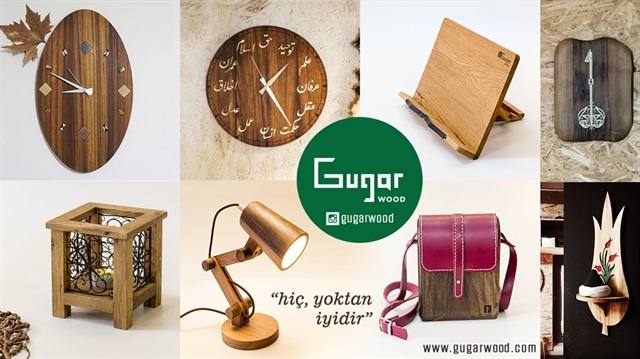This image appears to be an advertisement for Gugar Wood, a company specializing in wooden handcrafted products. The advertisement is divided into 8 squares, each showcasing a different wooden item. In the top left corner, there are two wooden clocks: one is oval-shaped with a leaf design next to it, and the other is a round clock, both featuring distinctive lettering. To the right, in the upper middle squares, there is an elegant lap desk and a decorative wooden plaque. The left square in the second row displays a cut-out lamp holder, followed by a lit wooden lamp with the text "H-I-C, Y-O-K-T-A-N" and "I-Y-I-D-I-R" punctuated beneath it. Next to it is a square featuring a wooden purse with a red leather top and strap, with the website www.gugarwood.com written nearby. The final square on the bottom row showcases a wooden sconce holder, possibly for incense, designed in a petal shape adorned with flowers. At the center of the advertisement is a large green circle with the company name "Gugar Wood" in white text and a logo below it. The Instagram handle "Gugar Wood" and the text www.gugarwood.com are also prominently displayed, along with a quote in a foreign language, possibly Dutch.